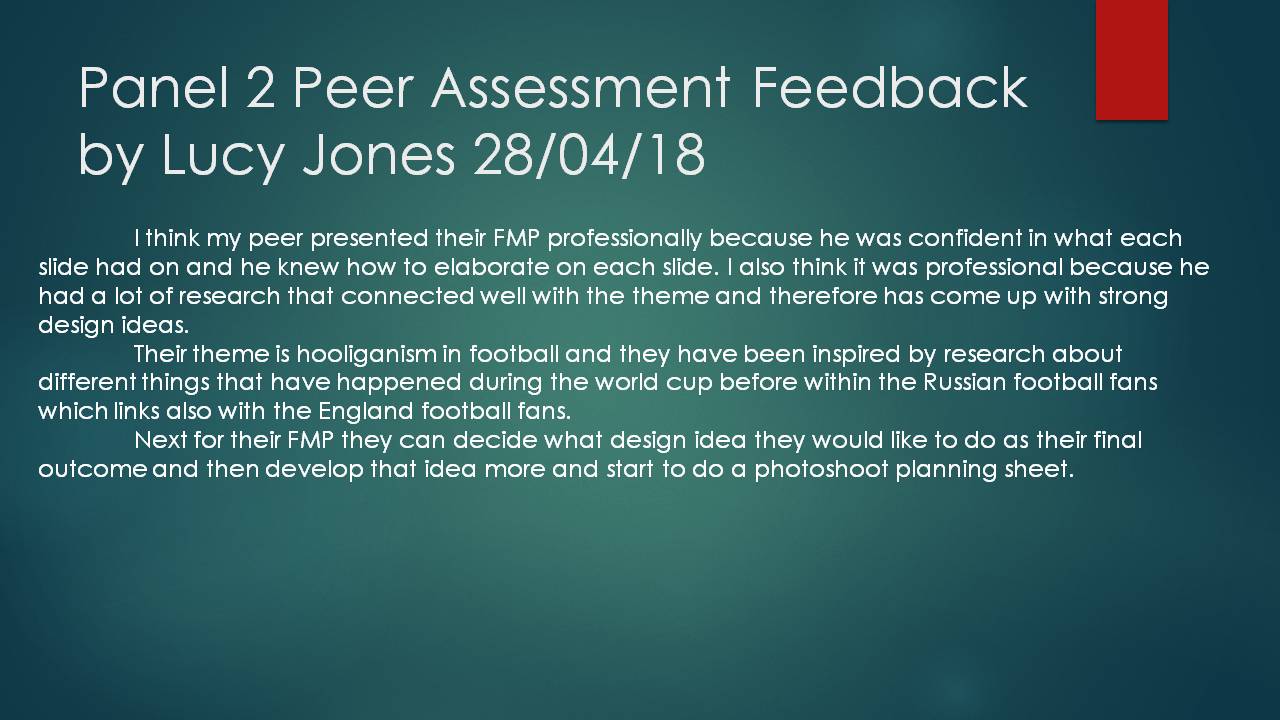This is an image of a PowerPoint slide with a background that transitions from dark greenish turquoise at the corners to a lighter shade in the center. In the top right corner, there's a small vertical red rectangle. The primary text, located in the top left, reads in large white font: "Panel 2, Peer Assessment Feedback by Lucy Jones, 28/04/18." Below this, in smaller white font, there's a detailed peer review stating: "I think my peer presented their FMP professionally because he was confident in what each slide had and knew how to elaborate on each slide. I also think it was professional because he had a lot of research that connected well with the theme and therefore has come up with strong design ideas. Their theme is hooliganism in football, and they have been inspired by research about different events that occurred during previous World Cups involving Russian and English football fans. Next, for their FMP, they can choose a final design idea to develop further and start planning a photo shoot."